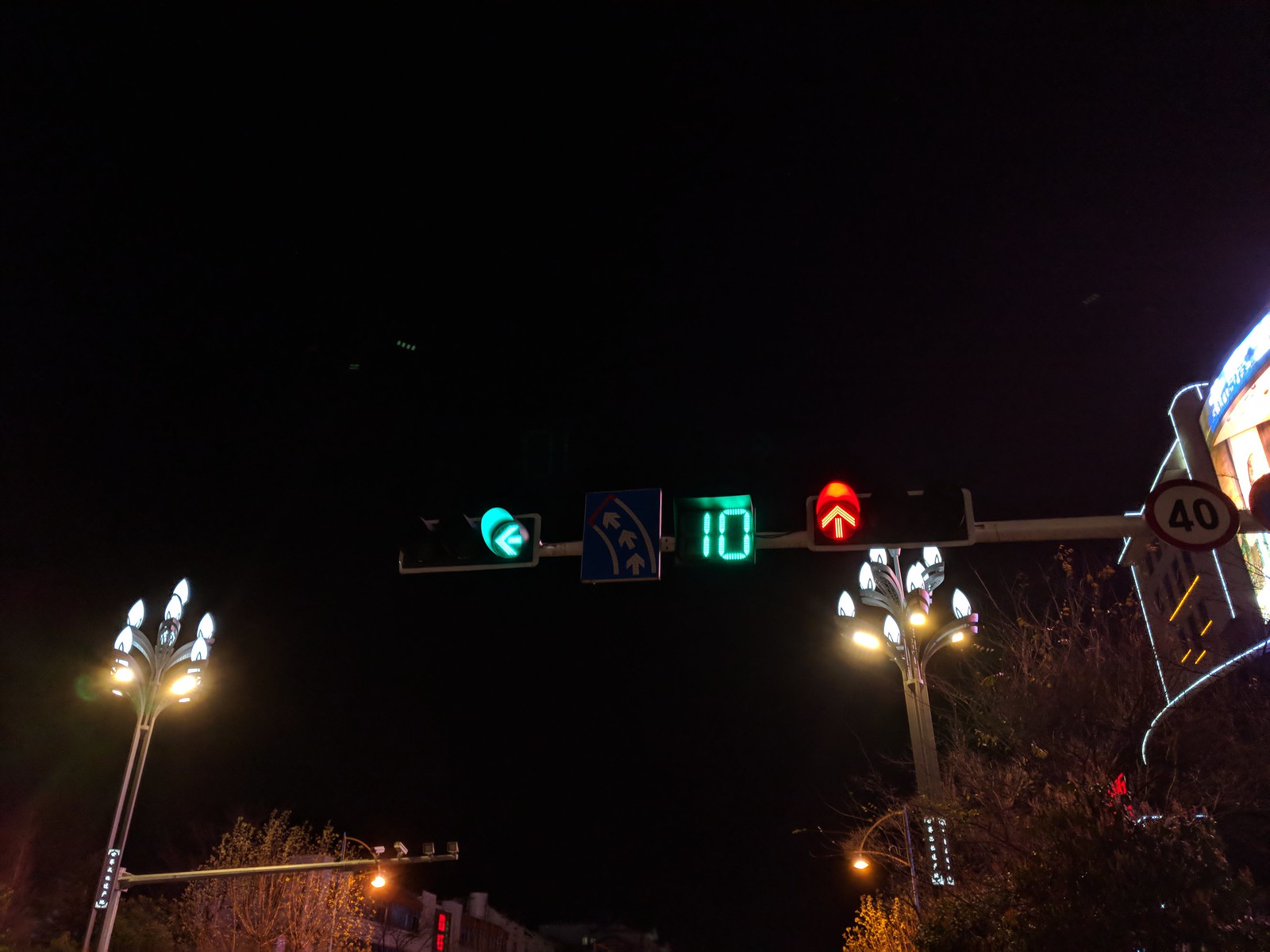The image captures a nighttime street scene beneath a dark, nearly black sky dotted with a few white stars. The camera is angled upwards, focusing on a pole laden with various signs and lights in the foreground. Central to the image is a traffic light displaying a mint green "10," flanked by a green light on the left and a red light on the right. Above these, a blue sign with white arrows directs traffic. To the right of the pole, there's a circular "40" mph speed limit sign. The background reveals a couple of street lights, adorned with multiple light fixtures reminiscent of candle tips or leaves on a tree. The scene also features the tops of a couple of buildings—one prominent on the right and another partially visible in the distance—adding depth to the dark backdrop. In the distance, a sign that seems to be for a theater is illuminated, contributing to the scattered, ambient glow in this otherwise dark nightscape.